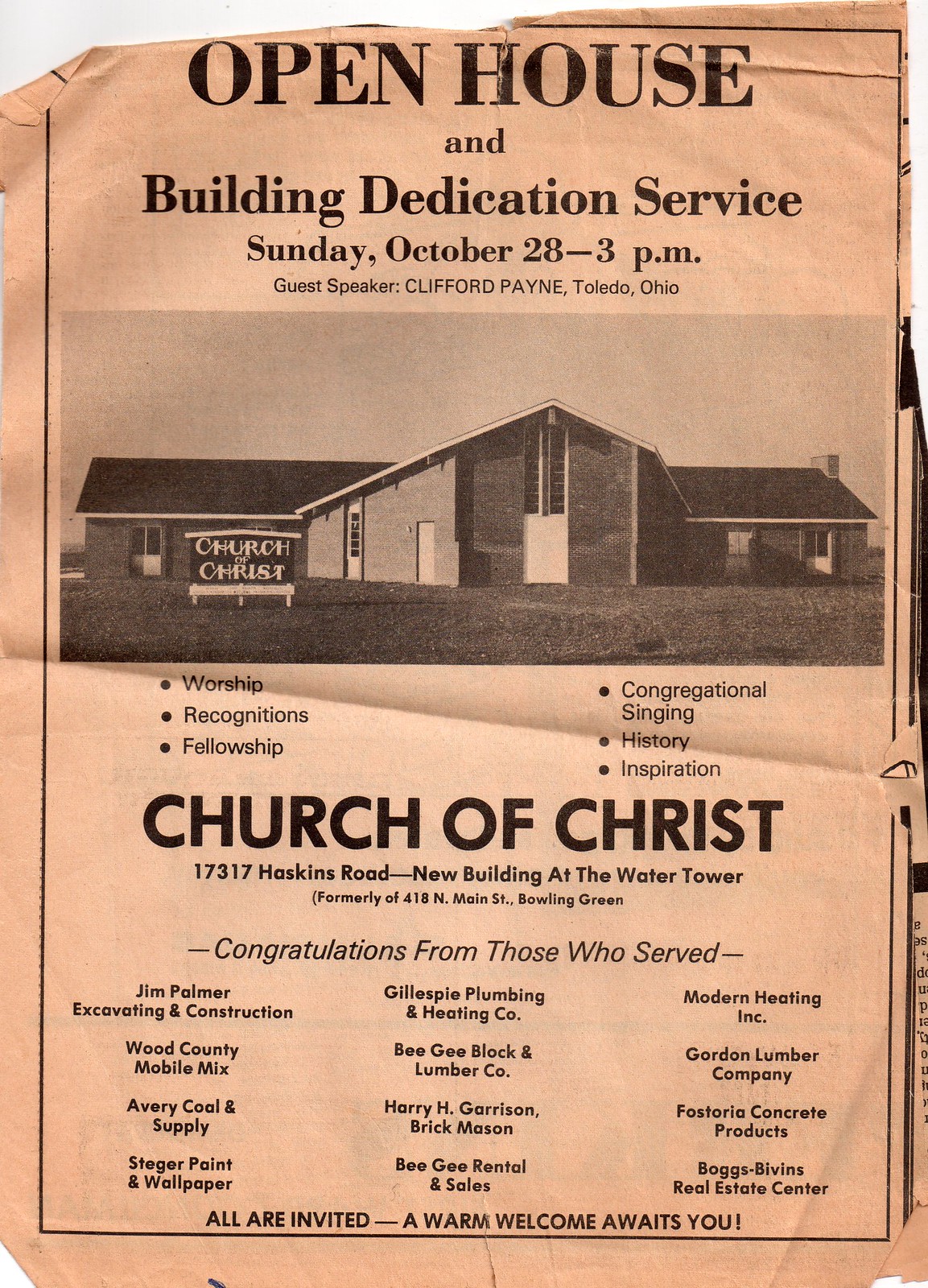This image portrays an old, slightly pink, and worn poster or possibly a folded piece of paper. The poster announces an open house and building dedication service for the Church of Christ, scheduled for Sunday, October 28th at 3 p.m., with guest speaker Clifford Payne from Toledo, Ohio. The top of the poster prominently displays the words "Open House," while further details about the event are provided below. 

In the center, there's a black-and-white picture of a modest, single-story church, with a black sign in front that reads "Church of Christ." This sign also lists the following activities and themes: worship, recognitions, fellowship, congregational singing, history, and inspiration. The address for the new building is 17317 Haskins Road, located at the Water Tower, previously situated at 418 North Main Street, Bowling Green. 

Towards the bottom of the poster, there's a section congratulating those who served in the church's construction, mentioning Jim Palmer Excavating and Construction, Gillespie Plumbing and Heating, and Modern Heating Incorporated, along with nine other businesses. The poster concludes with a warm invitation: "All are invited, a warm welcome awaits you."